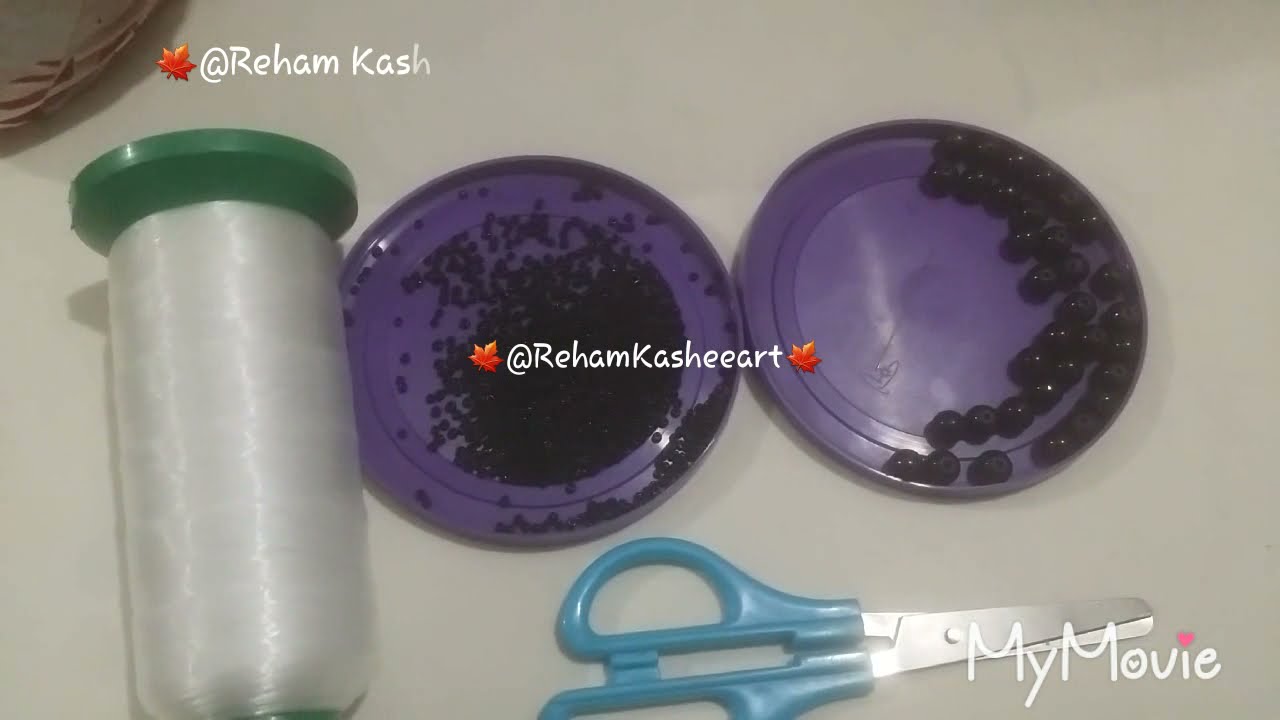Set against a white surface, the image features an assortment of objects. On the upper left, there is a test tube with a silvery surface and a green lid, which stands beside a small orange leaf labeled "Abraham Cash." Below the leaf is a spool of crystal thread commonly used for beading or making bracelets. Central to the image are two purple circular dishes: the left dish contains very small black beads, and the right dish holds slightly larger black beads. Between these dishes, there is another small orange leaf inscribed with "Abraham Cash Heart" and another leaf without text. At the bottom of the image, a pair of scissors with blue handles and silver blades is visible. Additional text reads "My Movie," and the colors in the image include brown, white, silver, green, red, purple, light blue, and pink. The setting appears to be indoors, possibly an arts room.